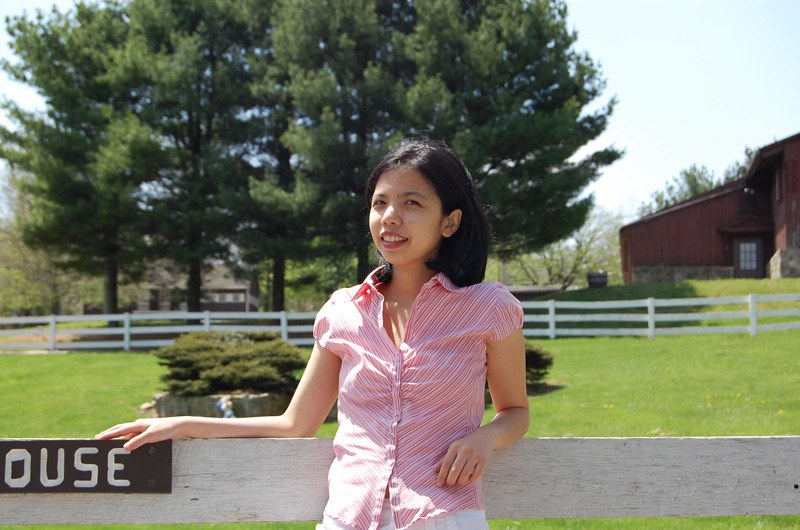The image captures a bright, outdoor setting in what appears to be a picturesque field during the day. The central focus is a slender, young Asian woman, likely in her teens, smiling warmly at the camera. She is dressed in a pink, short-sleeved shirt adorned with red, pink, and white stripes, paired with white pants. Her shoulder-length, black hair gently brushes her neck.

Leaning casually against a white fence, she adds a sense of calm and ease to the scene. The fence features a partially visible wooden sign that reads "O-U-S-E," suggesting the word "house." 

Behind her stretches a sweeping field dotted with bushes and bounded by another white fence, this one with horizontal rails. Further into the background, a dense stand of green trees adds depth to the idyllic setting. To the top right corner of the image, a brown building with a sloped roof stands against a backdrop of a vast blue sky with scattered clouds. The overall ambiance of the photo is serene and inviting, capturing a moment of tranquility in a rural landscape.